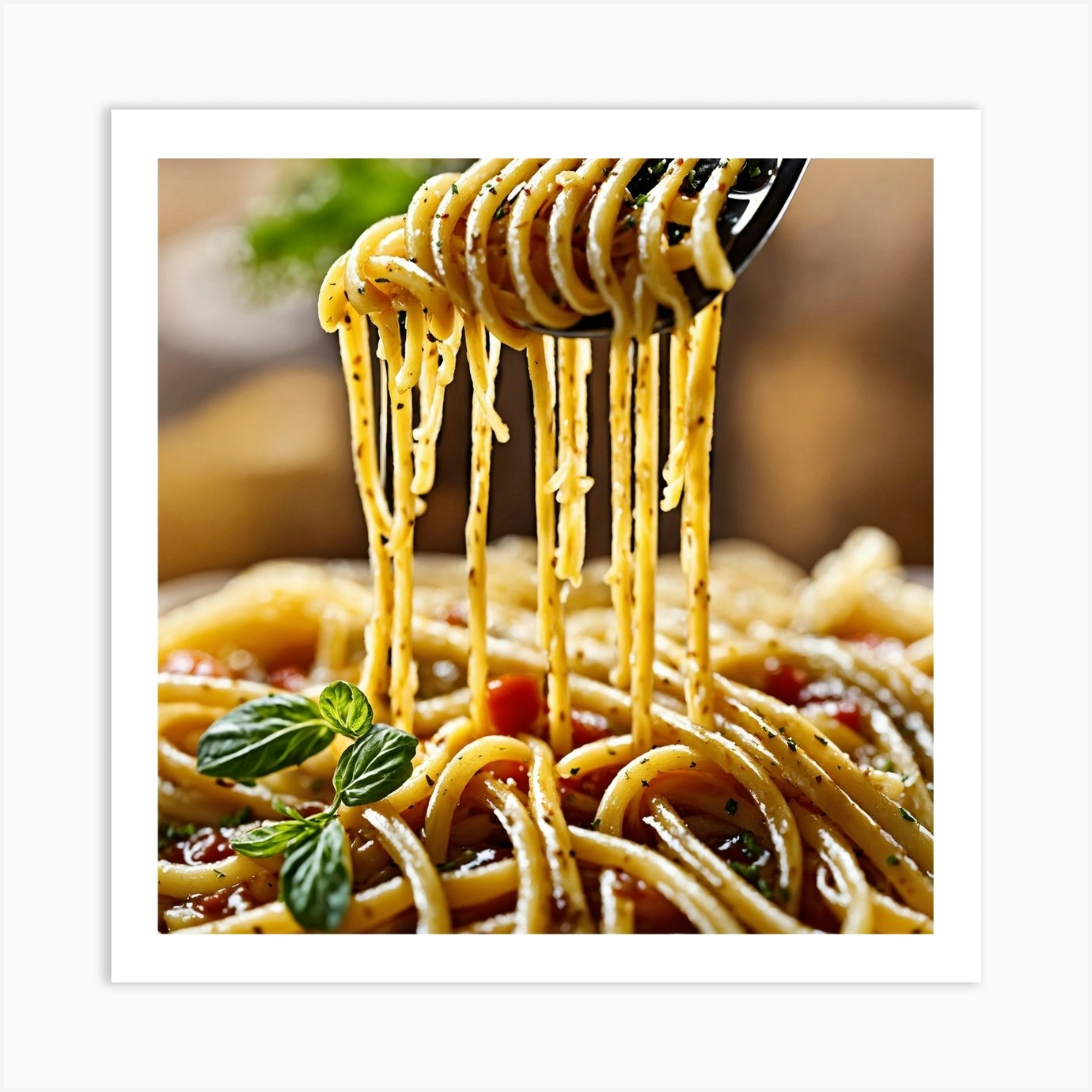A photograph bordered in white captures a utensil lifting a serving of spaghetti. Though it's difficult to ascertain if it is a fork or a spoon, it's performing the classic motion of twirling the spaghetti around its tines, causing long strands of pasta to dangle. The spaghetti is coated in a garlic butter sauce, devoid of marinara, allowing the glistening strands to reveal slivers of tomatoes interspersed throughout. A sprig of young basil adorns the dish on the left side, adding a touch of freshness. The pasta is lightly covered with butter or olive oil and sprinkled with black pepper, oregano, and other Italian seasonings, enhancing its flavorful appearance.